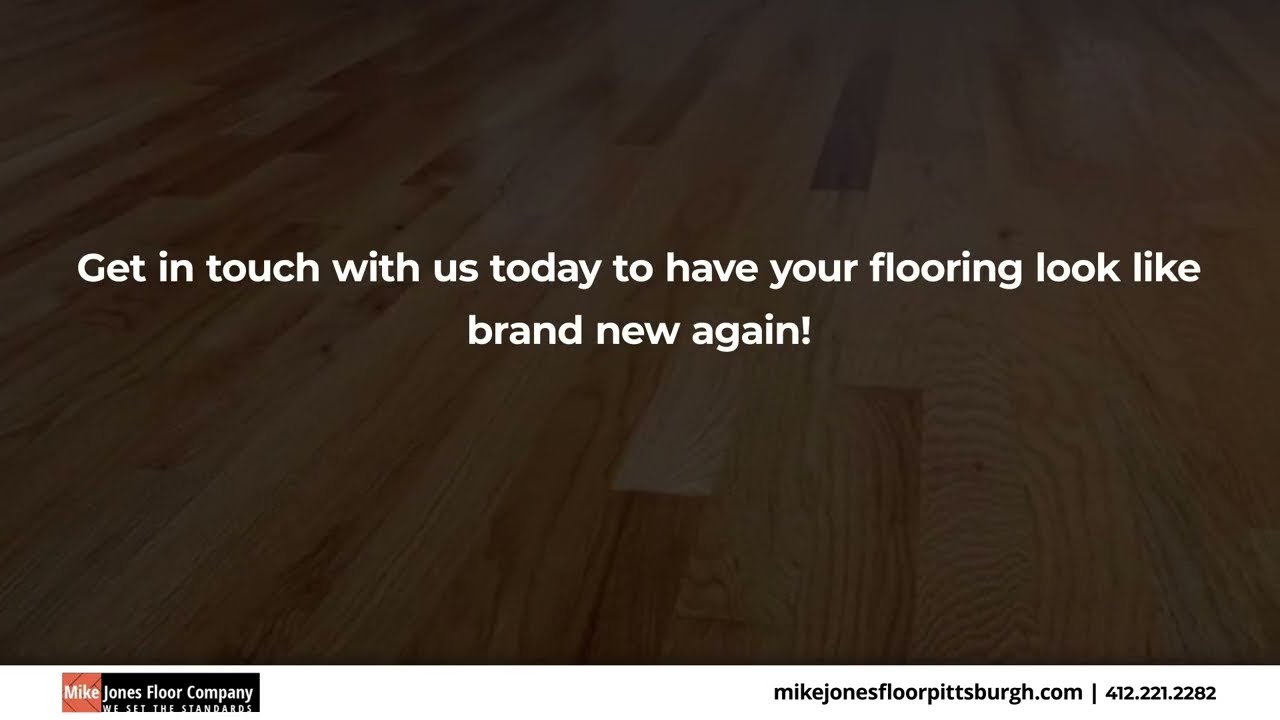This color advertisement for Mike Jones Floor Company features a landscape orientation with a dark, brown hardwood floor in the background, giving it a sleek and sophisticated look. The flooring is pictured in a dim light, enhancing the depth and richness of the wood grain. Prominently displayed in the center of the image, in crisp white sans-serif font, are the words: "Get in touch with us today to have your flooring look like brand new again!" The bottom section of the advertisement is divided into two parts: on the lower left, there's the company's logo—'Mike' in white letters on a red background and 'Jones Floor Company' in white on a black background with additional text; on the lower right, the contact details are clearly listed with the website, MikeJonesFloorPittsburgh.com, and the phone number, 412-221-2282. The overall design is a harmonious blend of photography and graphic elements, creating a polished and professional visual appeal.